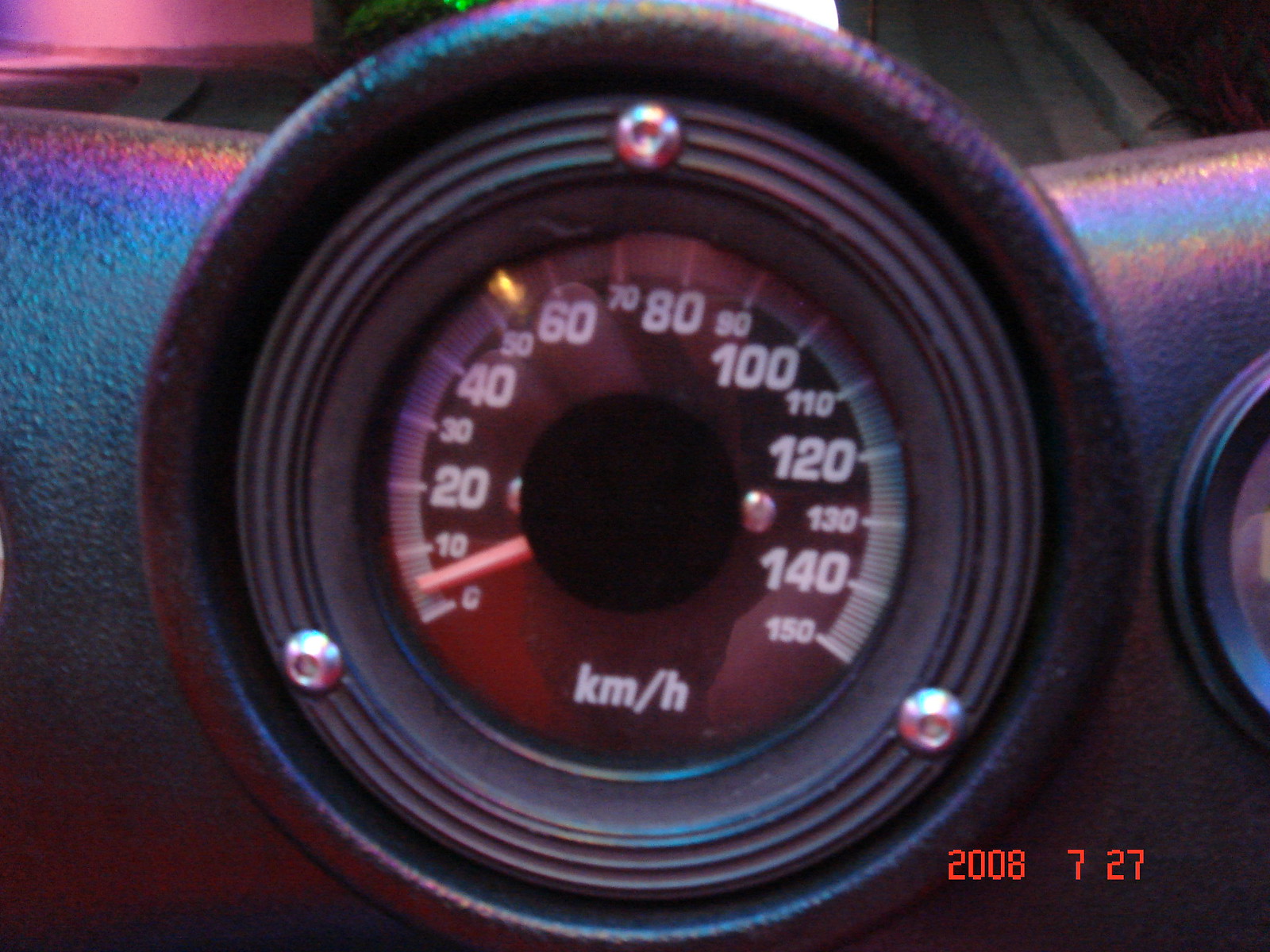This image showcases a close-up of an odometer, likely from a car or motorcycle, given the compact size of the speedometer. The speedometer displays values ranging from 0 to 150 kilometers per hour, with numerical intervals marked at every ten kilometers. Beneath the numbers, there is a label indicating "km/h." The bottom right corner of the image contains a date stamp, "2008-07-27," signifying that the photograph was taken on July 27, 2008.